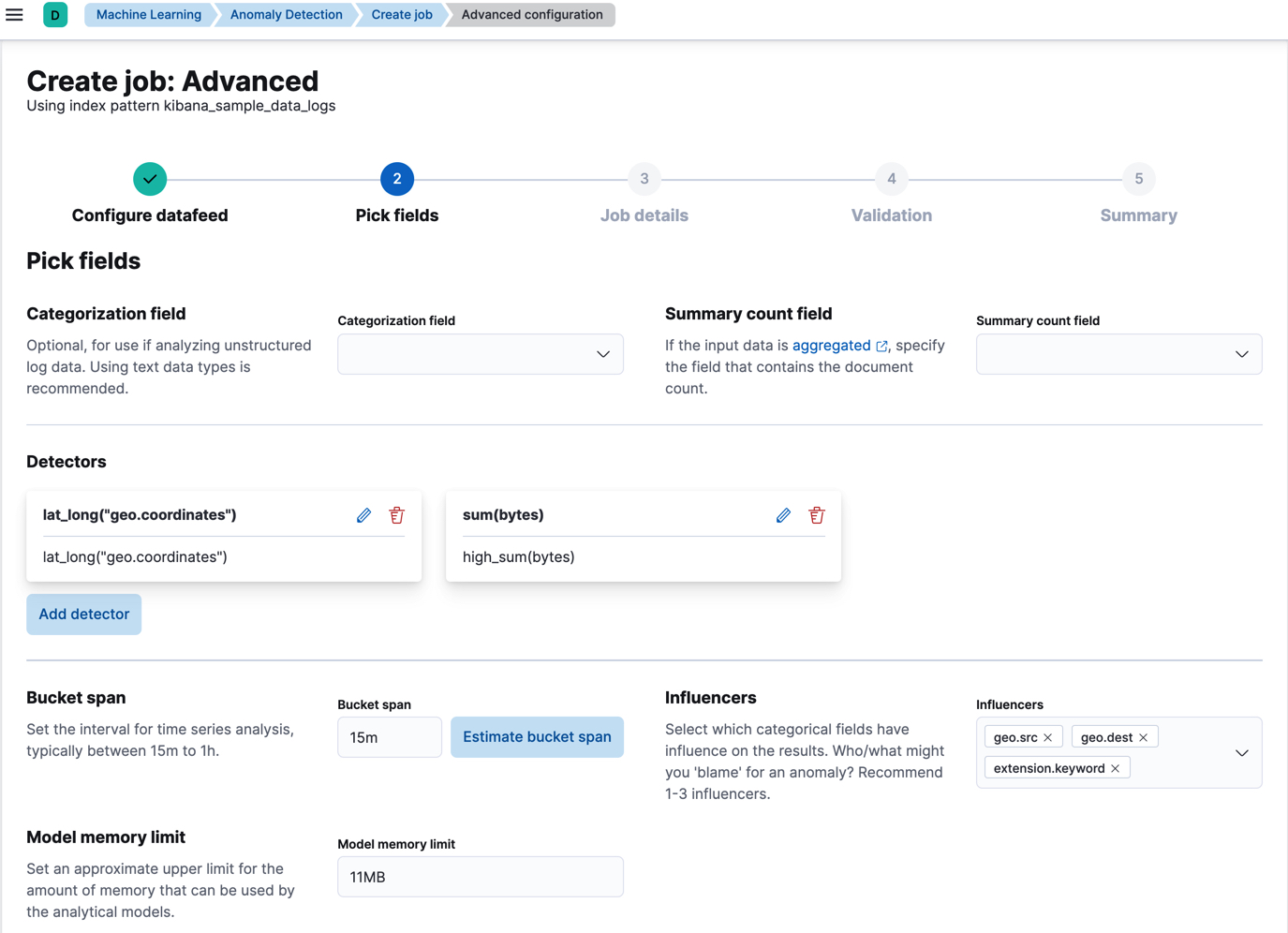The image appears to be a detailed interface for setting up a machine learning job in Kibana. At the top, there are three horizontal lines indicating a drop-down menu. Below that, headings are displayed in blue boxes shaped like arrows, including "Machine Learning," "Anomaly Detection," "Create Job," and "Advanced Configuration." 

In the "Create Job Advanced" section, the page makes use of the "Kibana Sample Data Logs" index pattern. A green circle with a checkmark indicates that data feed configuration is complete. To the right, a sequence of steps is displayed: 
1. A blue circle marked "Pick Fields,"
2. A gray circle for "Job Details,"
3. "Validation," and 
4. "Summary."

In the "Pick Fields" section, users see an option for "Categorization Field," which is optional and recommended for analyzing unstructured log data using text data types. A drop-down menu is available beside this field. Adjacent to it is another field labeled "Summary Count Field," also equipped with a drop-down menu.

The interface continues to the "Detectors" section, which includes an option to add detectors via a blue rectangular button. Beneath this, users can adjust the "Bucket Span," which is set to 15 minutes (15M). There is a button labeled "Estimate Bucket Span" for making time bucket estimations.

Further down, the interface includes options for setting "Influencers" and "Model Memory Limit," allowing for more granular control over the machine learning job configuration.